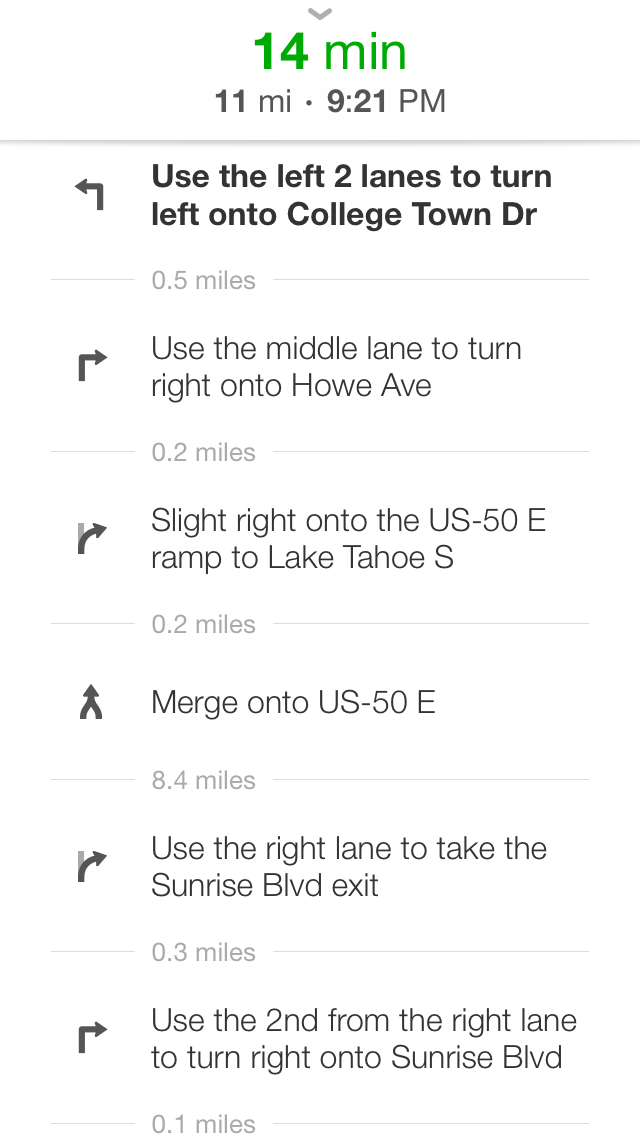In this image, we see a smartphone screen displaying navigation directions. At the top of the screen, there is green text indicating the travel time of 14 minutes. Directly below, in black print, it shows the distance of 11 miles and the current time, 9:21 PM. The directions are listed with corresponding arrows indicating each turn. The detailed route is as follows: 

1. Use the left two lanes to turn left onto College Town Drive.
2. Use the middle lane to turn right onto Howe Avenue.
3. Slight right onto the US-50 East ramp toward Lake Tahoe South.
4. Merge onto US-50 East.
5. Use the right lane to take the Sunrise Boulevard exit.
6. Use the second from the right lane to turn right onto Sunrise Boulevard.